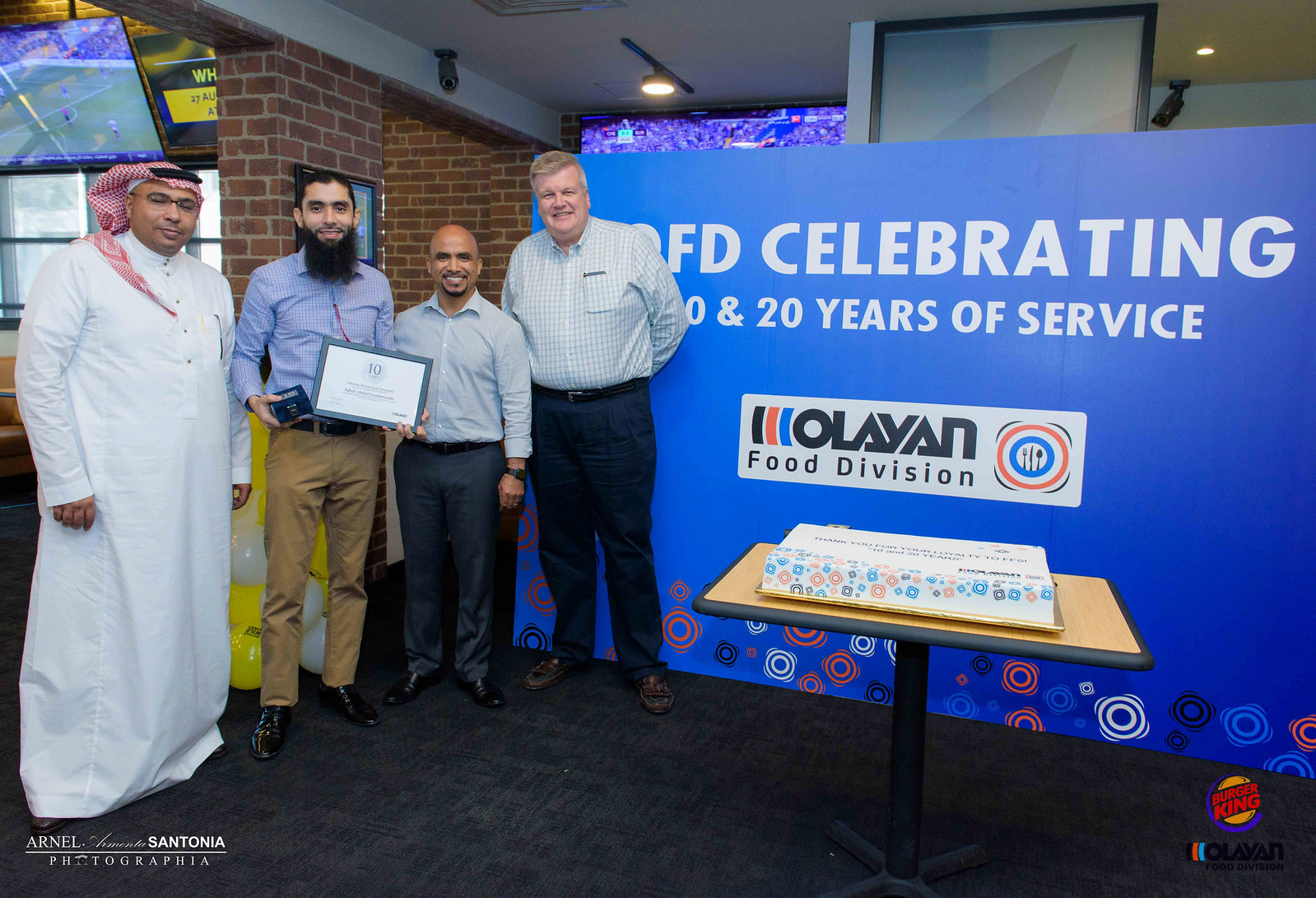The image depicts an indoor employee recognition event, possibly set in a warehouse or restaurant featuring brick walls, a white ceiling, and dark gray or black carpeting. Central to the scene is a large, tall blue sign stretching nearly from floor to ceiling. The sign is emblazoned with “Celebrating Over 20 Years of Service” and mentions "Olein Food Division" in a white rectangle. Near the bottom, the sign is decorated with red, blue, and black swirling designs.

To the right of the sign, a small pedestal table holds a cake decorated with similar swirling patterns. Standing next to the sign are four men, three who appear to be of Middle Eastern descent and one Caucasian man. One of the Middle Eastern men, who has a beard, is holding a placard or award, possibly the focus of the recognition ceremony. The men are dressed variably in traditional Arabic clothing and long-sleeved shirts with navy pants. In the background, big-screen TVs displaying sports games add to the celebratory atmosphere, suggesting a more casual or communal setting. There is an array of colors visible in the scene, including white, black, tan, blue, orange, pink, red, gray, and yellow.